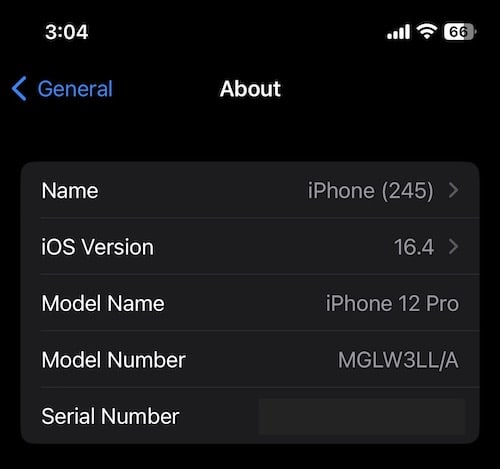A detailed partial screenshot of a mobile device's settings menu is displayed. The screen is outlined in black, providing a stark contrast to the lighter content inside. The status bar at the top shows the current time as 3:04, with a strong signal and active Wi-Fi. The battery icon indicates 66% remaining, with a white portion signifying the charged percent and a gray portion denoting the 44% yet to be charged.

Within the settings menu, the "General" option is selected and highlighted in blue, with a back arrow visible to return to the previous screen. The section titled “About” is displayed in white text. A light gray box below this section lists informational fields: Name, iOS Version, Model Name, Model Number, and Serial Number. Except for the Serial Number field, which awaits user input, all other fields are populated on the right side.